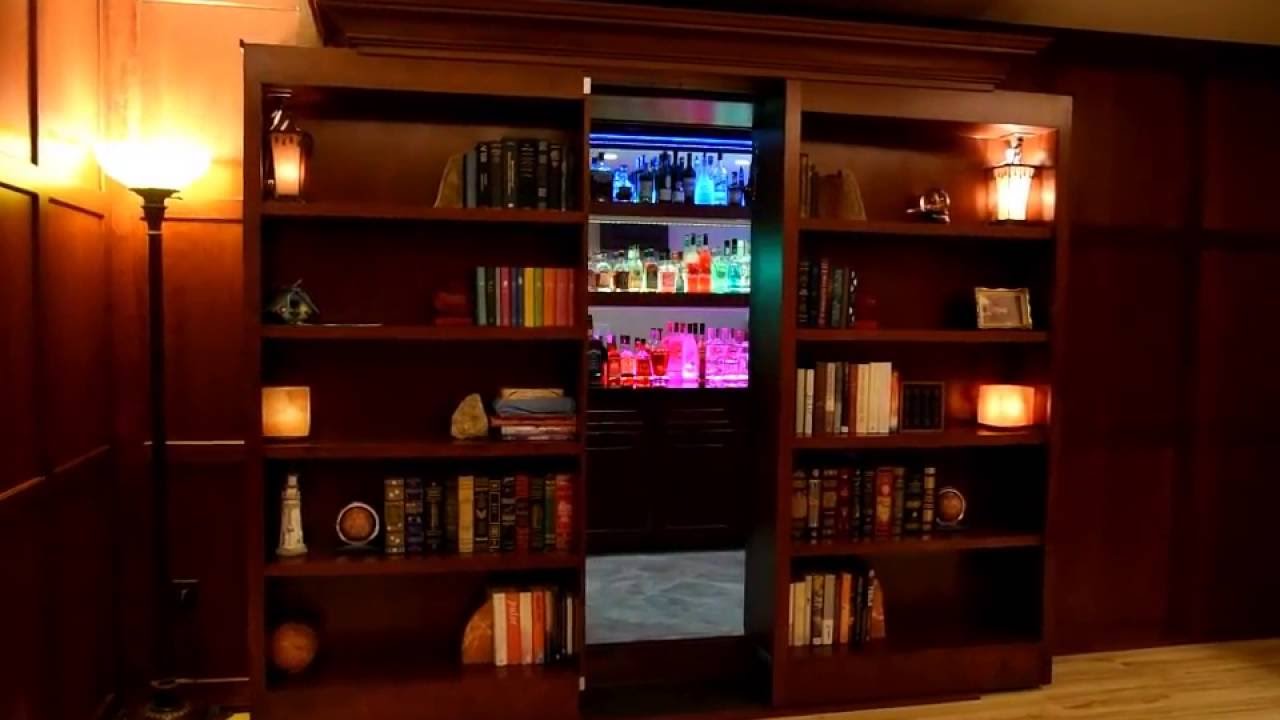The photograph captures an interior room featuring rich mahogany wooden paneling and a matching wooden floor. Situated in a den or an office, the room is dimly lit by a floor-length lamp in the left-hand corner, casting a soft glow on the surrounding paneled walls. Central to the image is an entertainment unit comprising three wooden bookshelves. The shelves are adorned with an eclectic mix of books, picture frames, and various trinkets. The most striking feature is the illuminated liquor cabinet in the center, showcasing a vibrant light display with three shelves holding bottles. The shelves emit a colorful glow—blue on the top shelf, transitioning to yellow-green, and pink on the bottom. Additional lamps atop the bookshelves contribute to the warm, subdued lighting that envelops the room, giving the photograph a cozy, intimate ambiance.